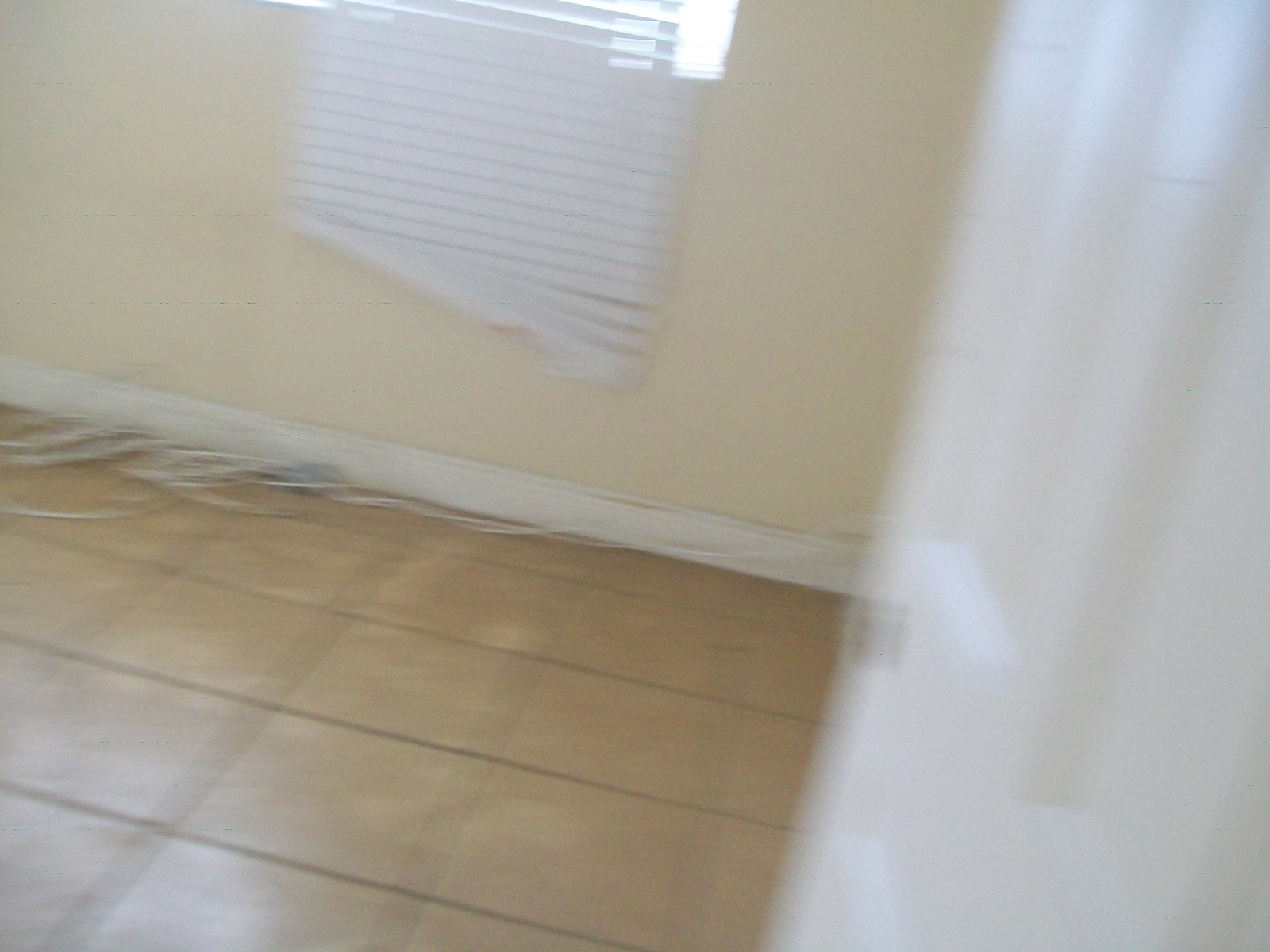This photograph captures the corner of a mostly empty room, possibly in a residential or commercial setting. Due to motion blur, the image lacks sharp focus and clarity. The room features brown mottled square floor tiles and white baseboards that line the base of buttercream-colored walls. In the corner where the baseboards meet the floor, a tangled pile of electrical cords is visible. Vertical blinds hanging lopsidedly on a window suggest they have been pulled too far from one side. In the foreground, there is a blurry door, likely indicating the point of entry into the room.